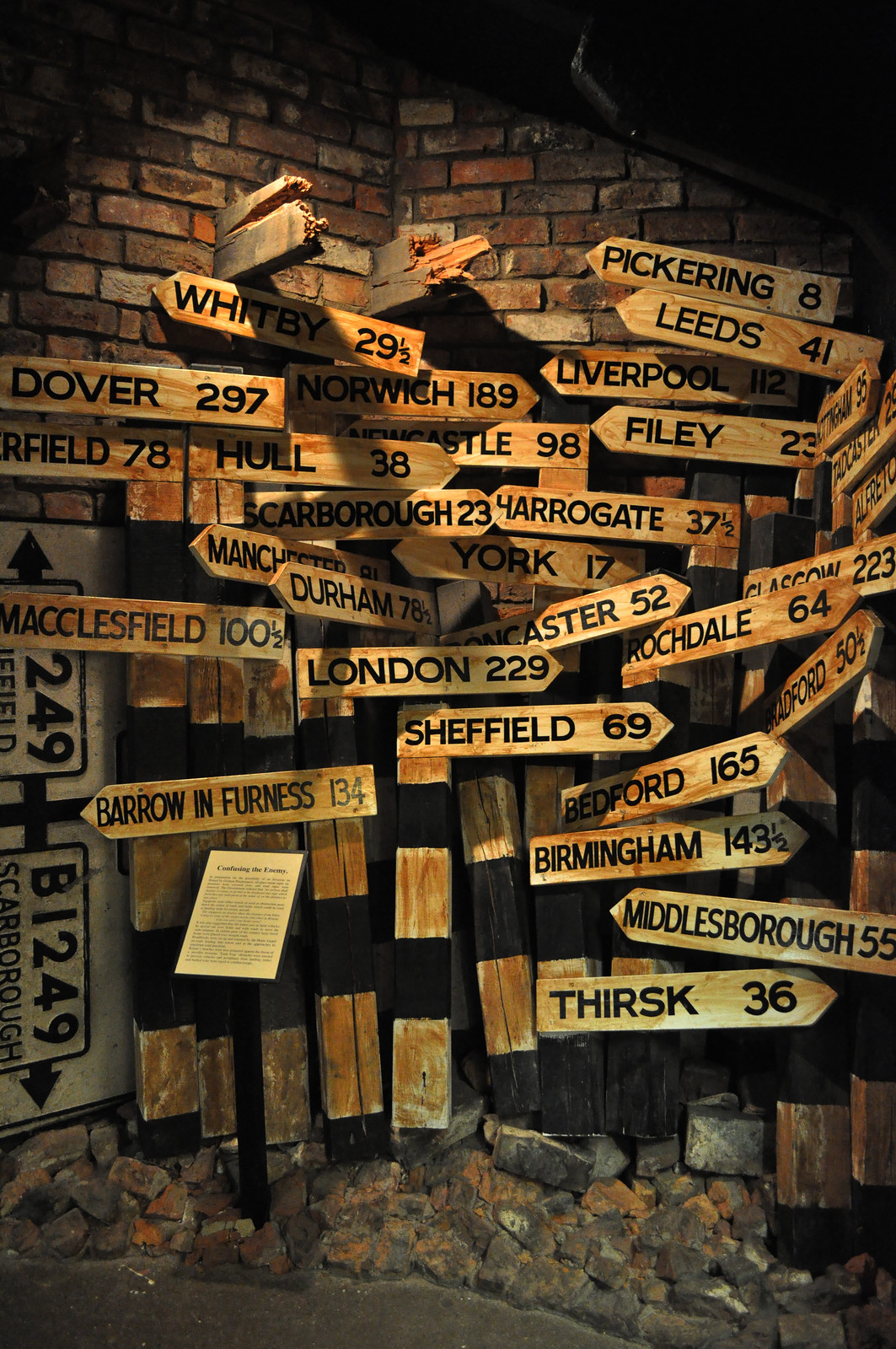The image portrays a dark corner where two brick walls intersect, forming a V-shaped nook illuminated by a single light. In front of these walls lies a collection of wooden street signs, each shaped like an arrow and listing various cities and their respective distances. The signs are densely packed, pointing in multiple directions—up, down, left, and right—creating a chaotic yet intriguing display. Some of the destinations include Sheffield 69 miles, London 229 miles, Filey 23 miles, Whitby 29.5 miles, Dover 297 miles, Macclesfield 100.5 miles, Barrow-in-Furness 134 miles, Rochdale 64 miles, Leeds 41 miles, and Yarrowgate 37.5 miles. Each sign is crafted in wood with black lettering, adding to the rustic and detailed aesthetics of the scene. Littered on the ground are pieces of brick, matching those of the walls but with no visible damage to indicate their origin. This image is either a drawing, painting, or computer animation and offers a curious blend of direction and disorientation within an urban environment.